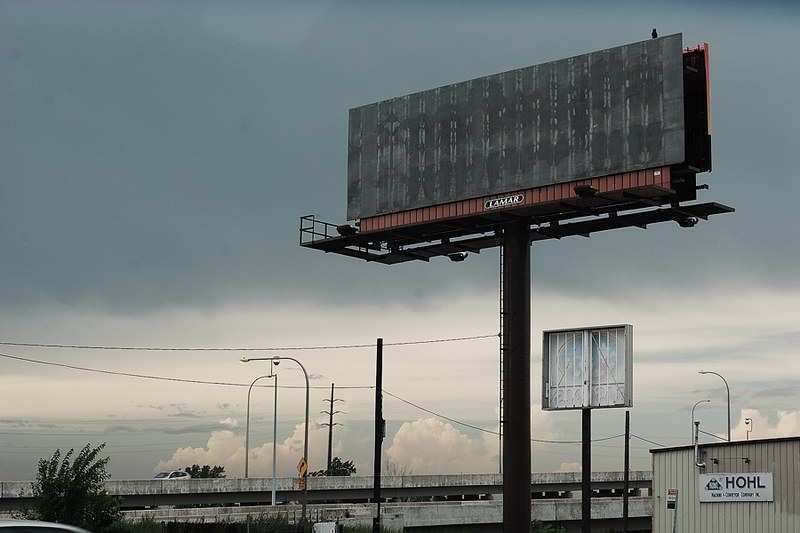An empty billboard, elevated on a sturdy, thick pole with a metal base, dominates the scene. The word "Lamar," likely indicative of the billboard company, is prominently displayed. Surrounding the billboard's front is a scaffolding structure, situated above a small office that bears the name "H-O-H-L." In the background, another smaller, also empty, billboard is visible. In the foreground, the top of a silver car comes into view, near silver lamp posts and yellow directional signs. Another car is seen, traveling down one of the streets. The sky is filled with puffy, gray clouds, contributing to the overcast ambiance. The scene includes three bushes and reflects an area that appears to have seen better days, hinting at a decline in vibrancy.